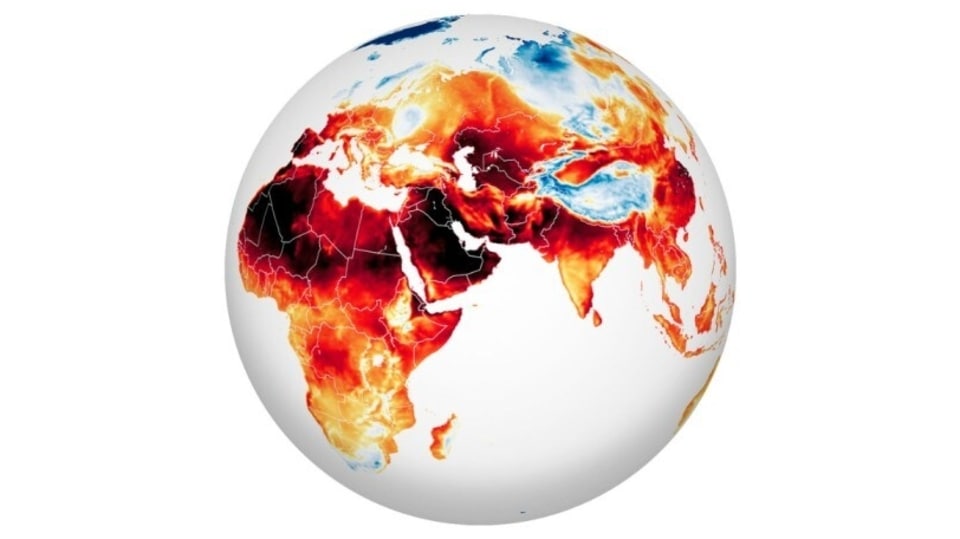This circular image portrays a highly stylized and color-coded photograph of the Earth against a stark white background. The oceanic regions are depicted in solid white, contrasting sharply with the landmasses, which display an intense gradient of colors. Africa, positioned on the lower left, transitions from green at its southernmost tip through yellow and orange, culminating in a dark red and almost black hue around the Sahara Desert. Adjacent to Africa, the Middle East, and Asia exhibit similar coloration, marked by vivid red and black tones. India, nestled between the landmasses, shows a progression from orange to red, terminating in black, while Europe displays a mix of orange and red, with Spain featuring notable black sections. The upper right section of the image incorporates areas of blue and light blue, suggesting water or perhaps cooler regions. Towards the north, distinct splashes of dark blue and light blue patches are mixed in, possibly indicating the Arctic waters. The overall fiery appearance, especially with pieces of land resembling flames and even dripping fire-like elements, emphasizes drastic climatic or environmental differences across the depicted regions.